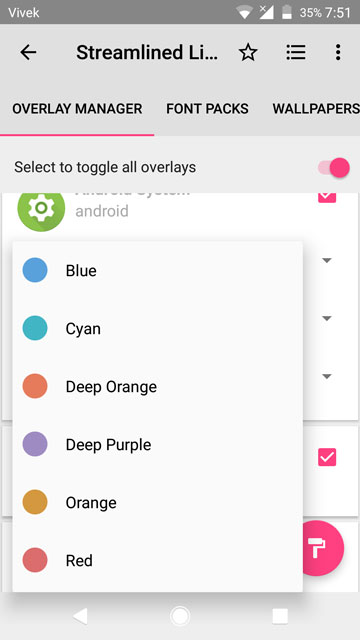**Detailed Caption:**

The screenshot depicts a smartphone interface with a dark gray status bar at the top. In the upper left corner, the name 'Bivek' is displayed, and on the right side, various status indicators are visible: a partially filled Wi-Fi signal icon, a fully filled carrier signal icon with an 'X' over it, indicating no service, and a battery icon showing 35% remaining. The time is displayed as 7:51.

Beneath the status bar, there's a navigation bar with a black arrow pointing left. The word 'streamlined' is partially visible in bold black text (“L-I…”), followed by a favorite star icon, a hamburger menu icon, and a three-dot menu icon.

The screen shows a list of options such as "Overlay Manager," "Font Packs," and "Wallpapers." A red line indicates the ability to scroll to see more options.

Below the list, the background lightens to a pale gray with a toggle bar labeled "Select to toggle all overlays," which is switched on in red. Additionally, there is a light gray box atop a white box displaying color options including Blue, Cyan, Deep Orange, Deep Purple, Orange, and Red in circular icons.

Further down, in a white area, there is a green circle with a white settings symbol, labeled 'Android' in gray text. On the right, part of a pink square with a white checkmark is visible. The interface also features three down arrows followed by a gray line, another pink box with a white checkmark, another gray line, and a pink circle with a white question mark.

At the bottom of the screen, the typical navigation buttons of a triangle, a circle, and a square are present.